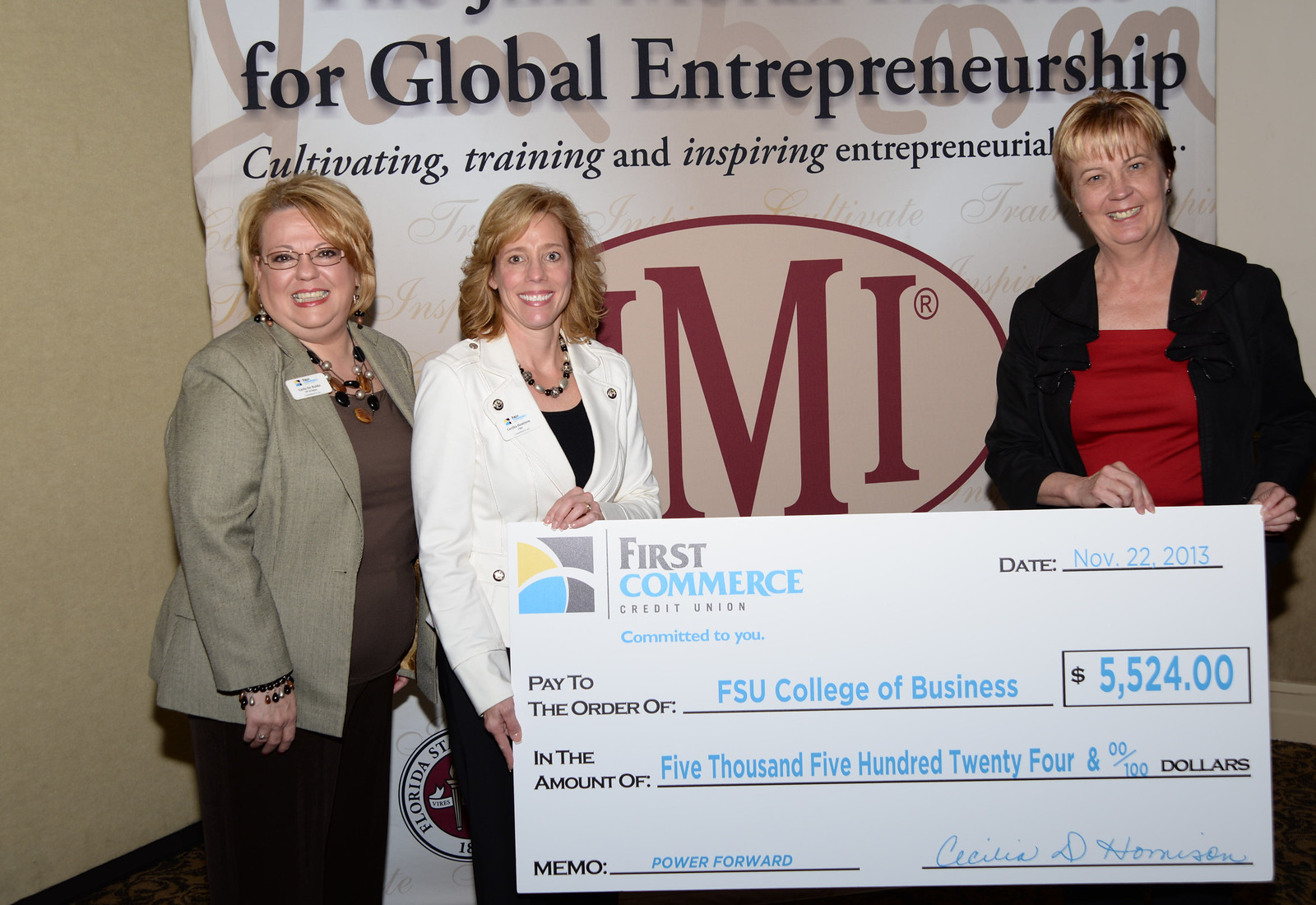The cool color landscape photograph captures three women standing in front of a backdrop that partly reads "for global entrepreneurship, cultivating, training, and inspiring entrepreneurial..." At the center of the image, two women are holding a large promotional check made out to the Florida State University College of Business for $524 from First Commerce Credit Union, dated November 22, 2013, with the memo "Power Forward." 

The woman on the left, dressed in a gray blazer, brown shirt, and black pants, wears glasses, a chunky necklace, bracelets on her right wrist, and a name tag on her blazer. To her right, the woman in the center sports a white suit coat over a black dress, a black and silver chunky necklace, and a name tag on her right side. The third woman, on the far right, has short blonde hair with bangs, a black jacket, and a red shirt. All three women share blonde hair and are smiling for the camera, creating a vibrant display of unity and celebration at the global entrepreneurship event.